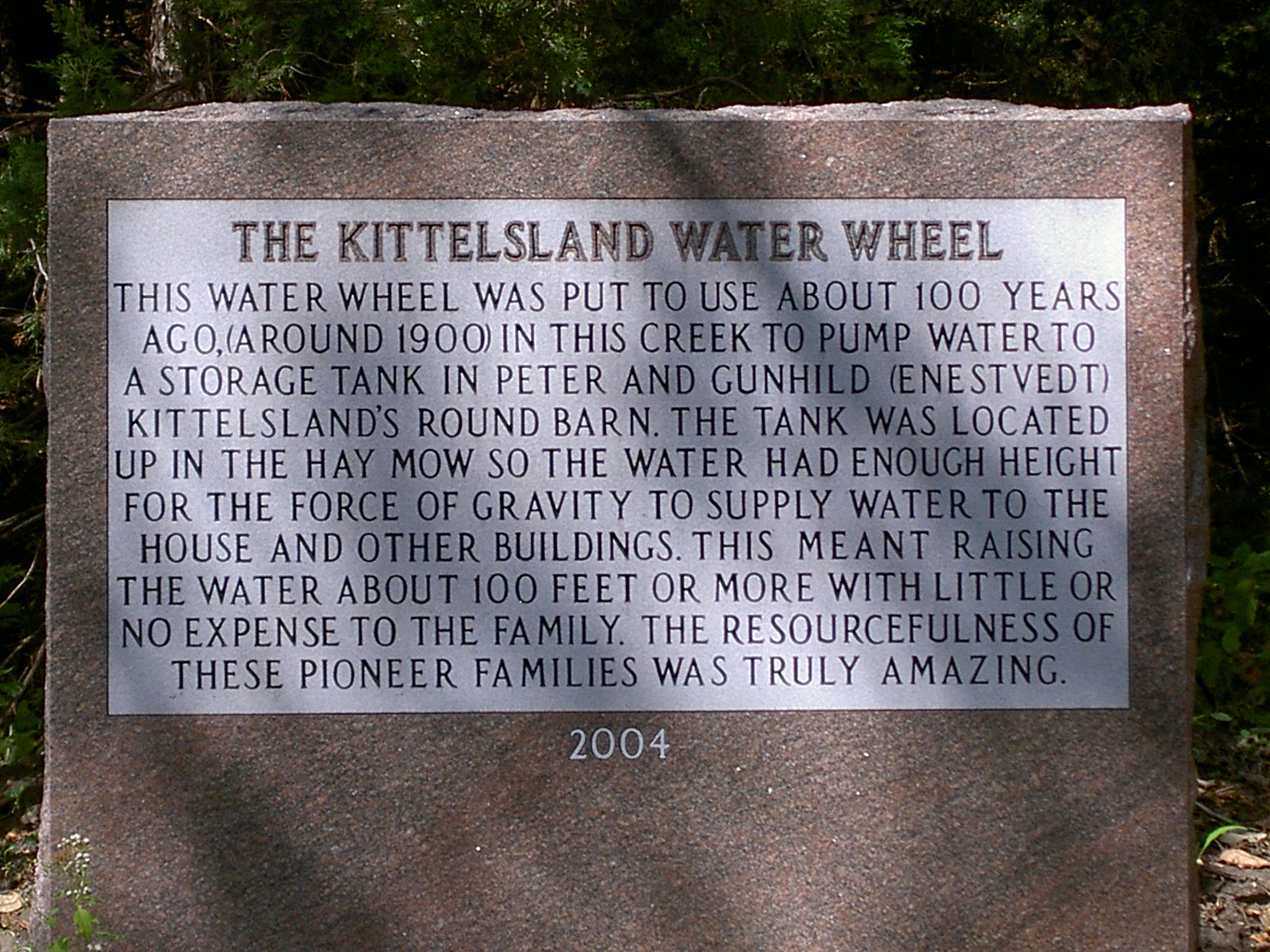The image features a substantial rectangular stone marker, which serves as a memorial plaque for the historic Kittlesland Waterwheel. Crafted from dark brown stone, this marker prominently displays an inscription on a gray square with black text. At the top, bold lettering announces "The Kittlesland Waterwheel." The detailed description below commemorates the innovative use of the waterwheel approximately 100 years ago, around 1900. This waterwheel was instrumental in pumping water from a creek up to a storage tank located in Peter and Gunnhild Kittleson's barn. Positioned in the hay mow, the tank's height, about 100 feet or more, enabled gravity to efficiently supply water to the house and other buildings without significant expenses. This ingenuity highlights the remarkable resourcefulness of the pioneer families in the area. The plaque, likely added in 2004, is situated against a backdrop of grass, soil, and possibly evergreen trees, evoking a sense of the natural environment where this historic innovation took place.